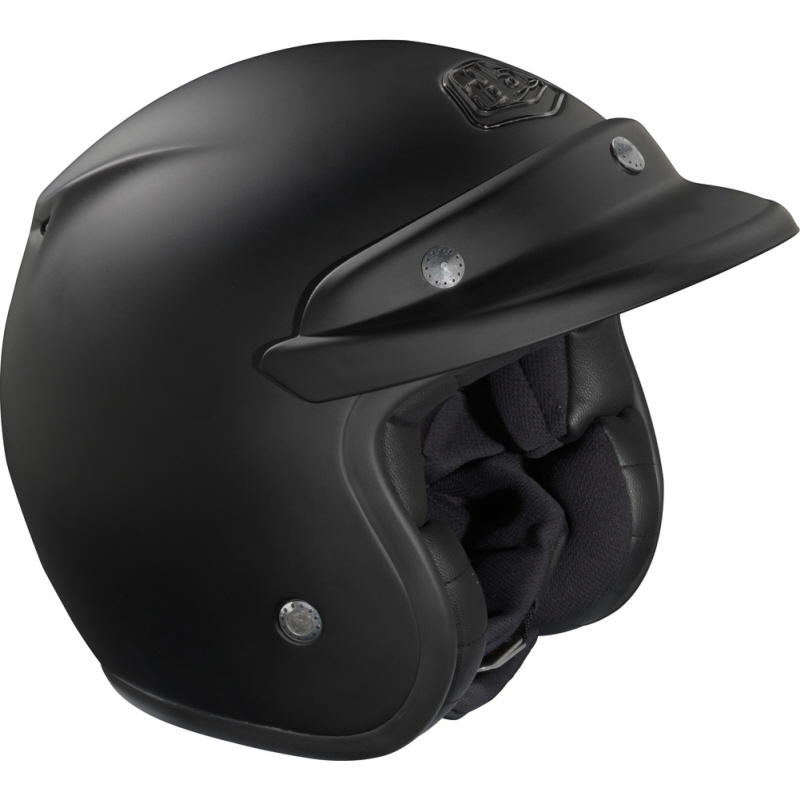The image depicts a sleek, all-black motorcycle helmet that appears to float against a white background, offering a detailed view primarily from the right side but with a slight angle showing a bit of the front. The helmet features a black visor adorned with two circular silver screws or buttons on each side. Over the forehead, there's an extra piece acting like a small brim to shade the eyes. Notably, the right ear area also displays a similar silver circular screw or button used for attachment. At the crown of the helmet, just above the visor, there is an embedded logo, though its specific design is indistinct. The inner padding, which looks quite cushiony and comfortable, is visible and appears to cover the ears and inner surfaces, providing adequate comfort. Additionally, a subtle design detail includes a concave or patterned indentation on the top left back of the helmet, adding to its sleek appearance. The helmet's matte black finish contrasts subtly with the silver accents, creating a modern and streamlined profile.